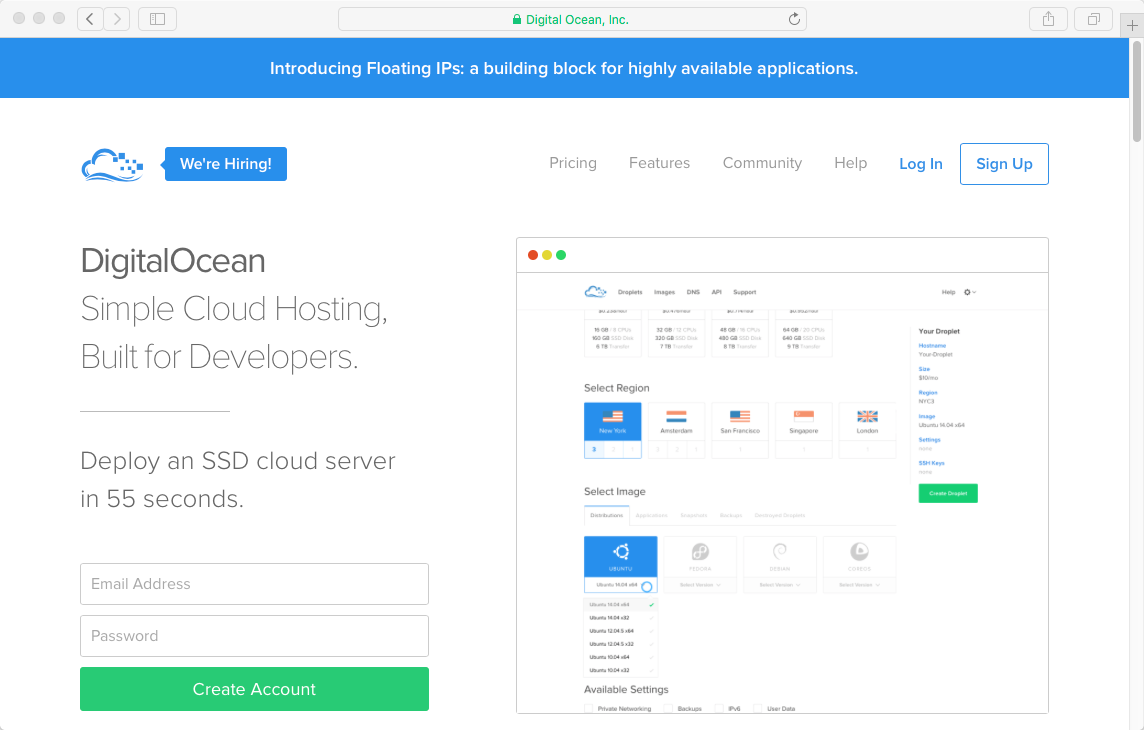A screenshot of the Safari browser displaying the DigitalOcean Inc. webpage. The interface includes a back button, forward button, home button, and a refresh button along the top. A prominent blue navigation bar at the top of the page displays the title "Floating IPs - A Building Block for Highly Available Applications". Beside it, a "We Are Hiring" button is visible.

Towards the bottom left, the page promotes DigitalOcean’s cloud hosting services with the tagline: "Sample cloud hosting built for developers. Deploy an SSD cloud server in 55 seconds." Below this, there's an option to input an email address and password, accompanied by a green "Create Account" button with white text.

At the top of the page, several navigation options are listed, including "Pricing", "Features", "Community", and "Help". There's also a blue "Login" button and a "Sign Up" button with a highlighted blue square.

Additionally, another section of the screenshot displays options for selecting server regions, though the text is small and difficult to read.

This webpage is a hub for DigitalOcean’s cloud hosting services, aimed at developers who need efficient and reliable hosting solutions for applications, including support for video game software development.